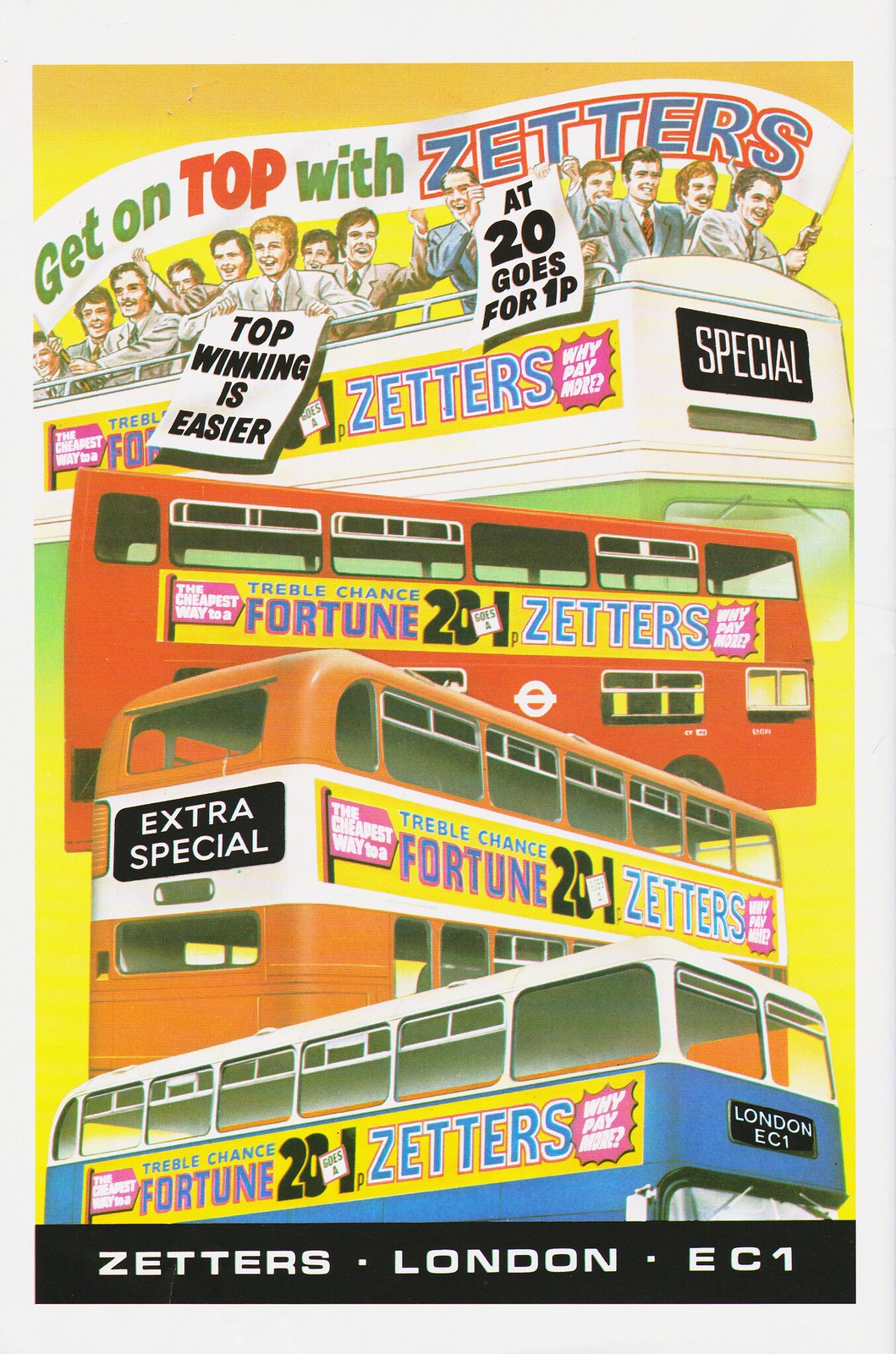The image is a colorful and vibrant print advertisement for Zetters, targeted at a British audience. Set against a bright yellow background with a white border and a black bottom border that reads "Zetters London EC1", this visually striking ad features a stack of four buses, one atop the other.

At the base is a blue and white bus adorned with banners that read "Fortune 21 Zetters", "Why Pay More", "London EC1", "Treble", and "Chance". Above it, an orange and white bus carries similar messages, including "Extra Special", "The Cheapest Way", "Treble", and "Chance". Next is a red bus, advertising "Treble", "Chance", "Fortune 21", and "Zetters Why Pay More". Finally, a white and green bus crowns the stack, with banners proclaiming "Special Zetters".

Atop the highest bus, a group of well-dressed, cartoon-like figures hold signs that state "Top winning is easier" and "At 20 goes for 1p". A prominent banner above them reads "Get on top with Zetters". The composition emphasizes the affordability and winning potential offered by Zetters, making it a dynamic and engaging advertisement.